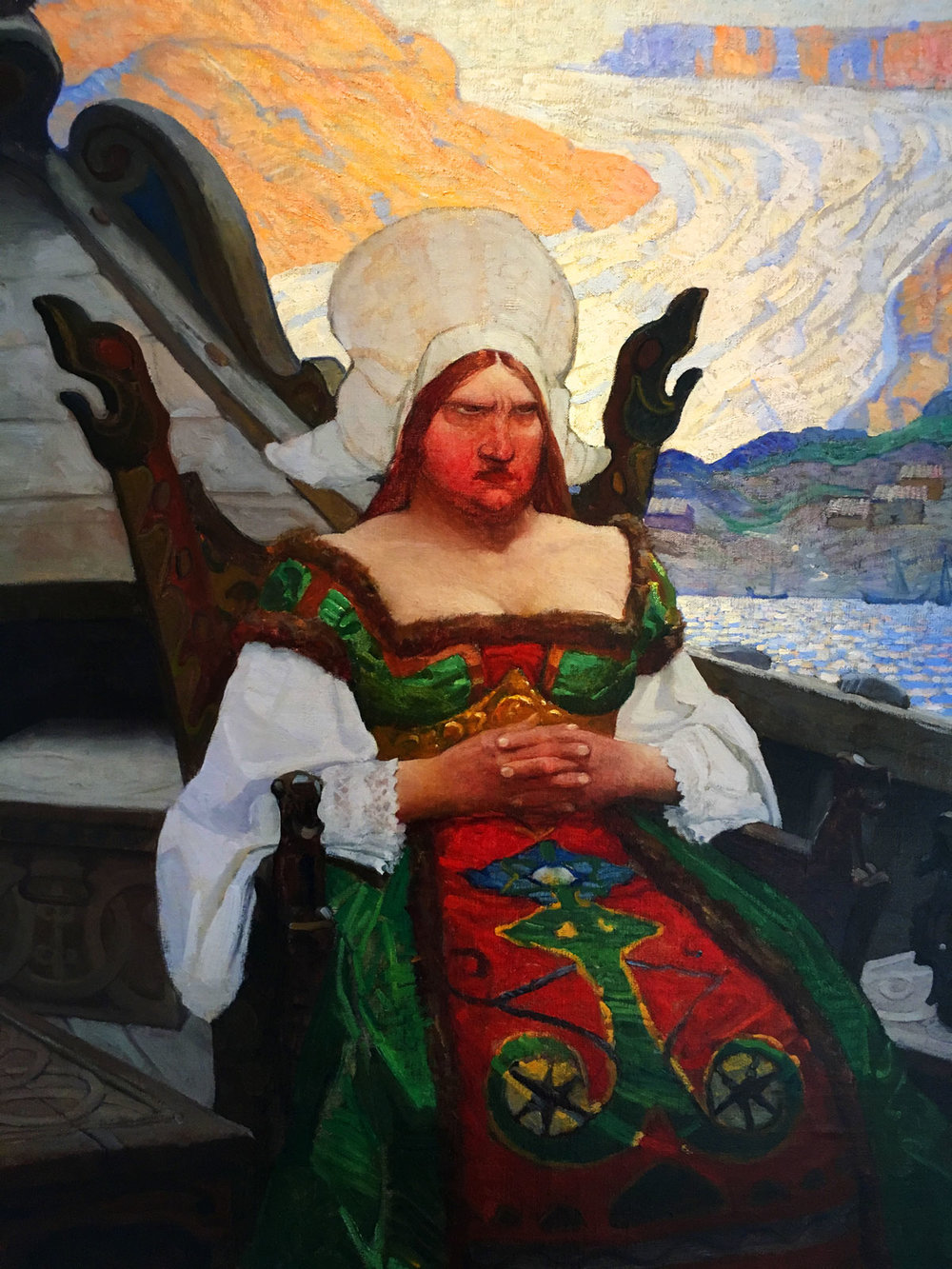This painting vividly depicts an angry-looking woman with a deep scowl, her intense features almost giving her a masculine appearance. She is seated in an ornate brown wooden chair that is adorned with spiked, alligator-like posts on either side. The woman dons a very detailed, pre-Victorian era dress, predominantly green with red accents and an anchor-like decorative design in the middle. The white sleeves are trimmed with lace, and she wears a high, Dutch-style white bonnet. Her long brownish-red hair frames her face. 

Her hands are neatly folded across her waist, displaying a shiny gold belt and intricate blue and gold designs down the middle of the dress. The chair appears to be situated on a wooden ship that resembles a Viking vessel, with visible rails and the peak of the ship's rear section. Behind her, there is an ocean with blue waters, a hillside featuring a couple of buildings, and a sky that is painted in orange, peachy, and white colors. The atmosphere surrounding the woman is both dramatic and detailed, emphasizing her displeasure and the intricate craftsmanship of her attire.